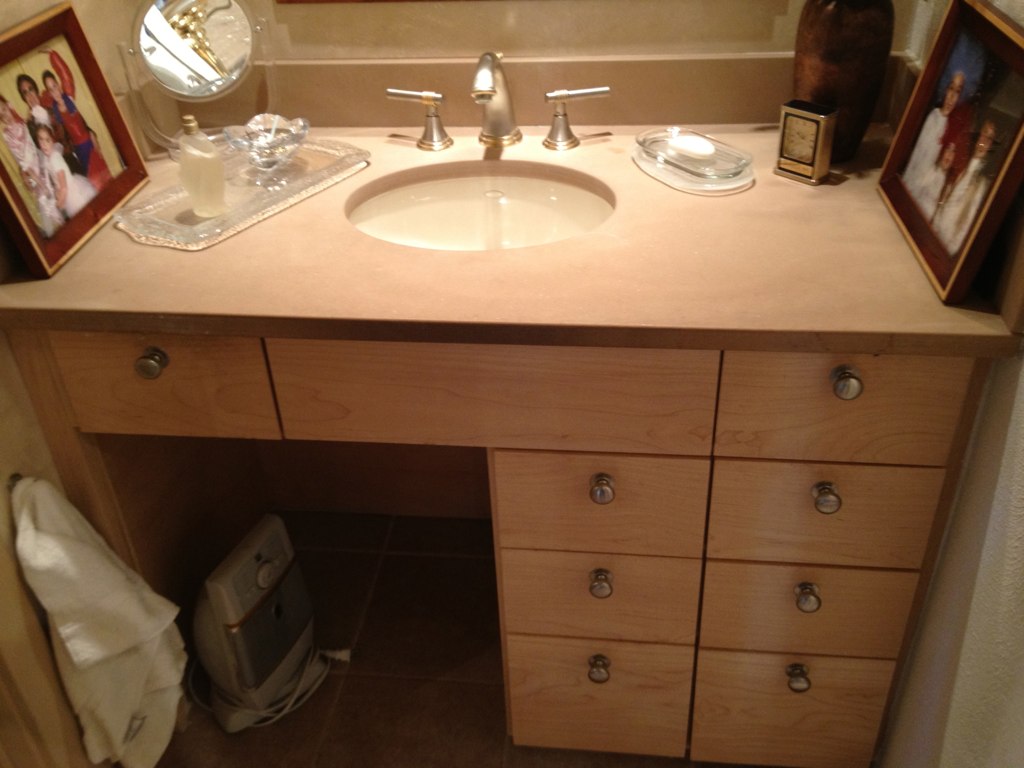This photograph, likely taken in the 1980s, depicts a bathroom dominated by a pinkish color palette. Central to the scene is a wooden vanity with a light-grained, potentially maple, finish. The vanity features an array of storage solutions: two drawers flanking either side of the sink, three additional drawers in a stacked configuration on the right, each adorned with a round silver knob, likely nickel-plated. This metallic accent is mirrored in the sink's fixtures, creating a cohesive look.

On the right-hand side of the sink, there is a clear glass dish holding a white Dove soap. Adjacent to this is a small, rectangular silver clock, solidifying the era as the 1980s with its vintage design. Beyond the clock stands a large, possibly glass or brown-colored vase. The vanity is complemented by a matching backsplash in the same linoleum texture and hue.

To the left of the sink, a larger glass dish showcases a clear perfume bottle, accompanied by a delicate rose petal-shaped bowl, perfect for holding jewelry. A vanity mirror, suitable for makeup application, stands beside these items. 

The bathroom is further personalized with framed photographs. One on the right side depicts three individuals in white attire with long hair, while another on the left features a man and three children possibly in Halloween costumes—a girl in a tutu and a colorful, acrobat-like costume on the right-hand side figure. 

Beneath the vanity, a white space heater with a wrapped cord is visible, indicative of the practical aspects of the room. In the bottom left corner, a small towel is neatly hung on a knob, adding a touch of everyday utility to this nostalgic snapshot of a meticulously detailed 1980s bathroom.